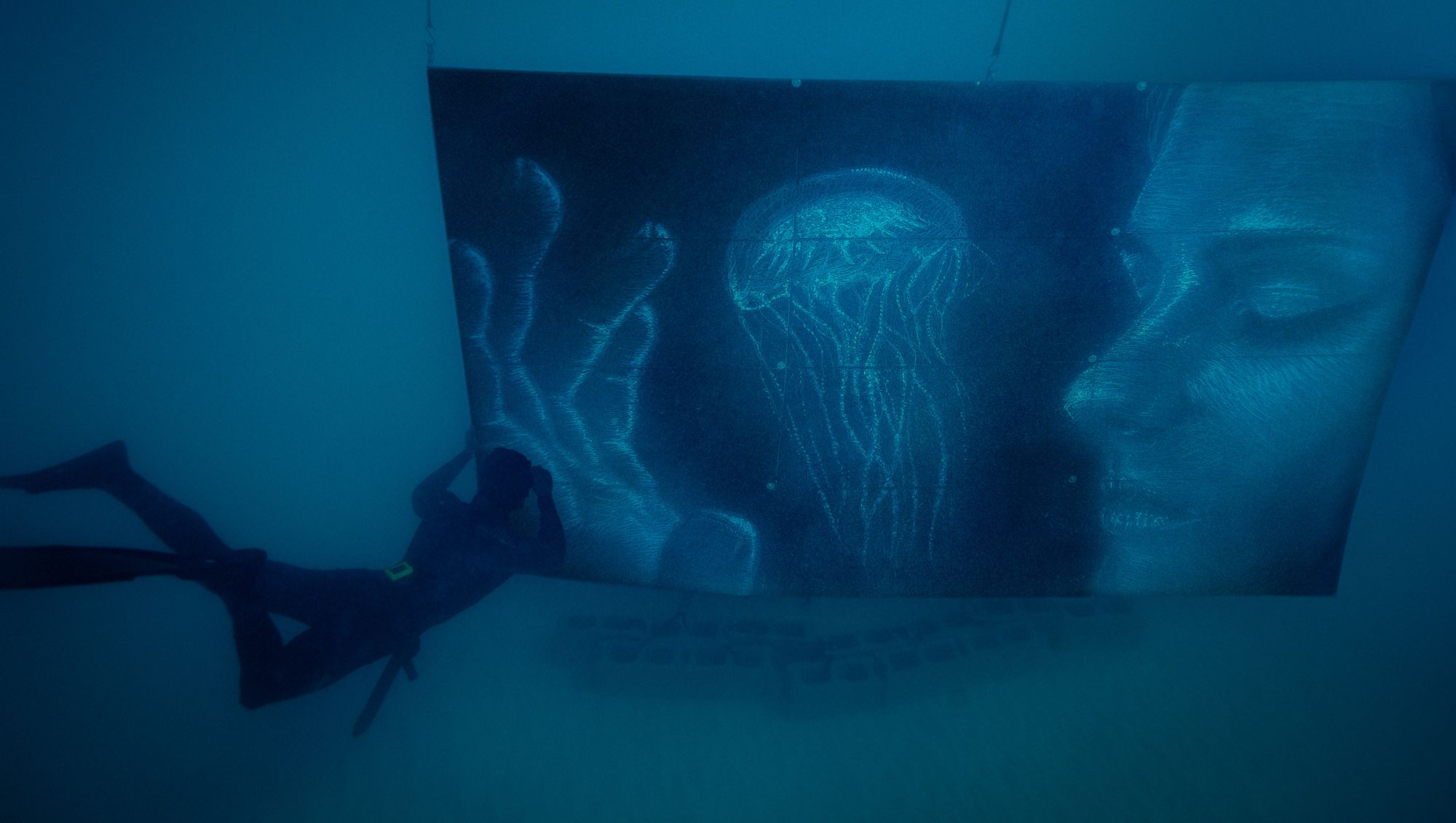The underwater scene captures a scuba diver positioned in the bottom left corner, appearing to interact with a large, blue-tinted billboard anchored to the ocean floor by cinder blocks. The billboard features a cyan-colored artistic portrayal of a serene woman's face with closed eyes, partially obscured by a large hand, creating a gap through which a jellyfish swims, its tentacles cascading down. The entire scene is enveloped in varying shades of blue and cyan, enhancing the ethereal ambiance of the underwater environment. The diver, equipped with flippers and diving gear, adds a sense of scale, emphasizing the billboard's imposing size against the dark, enigmatic backdrop of the ocean.